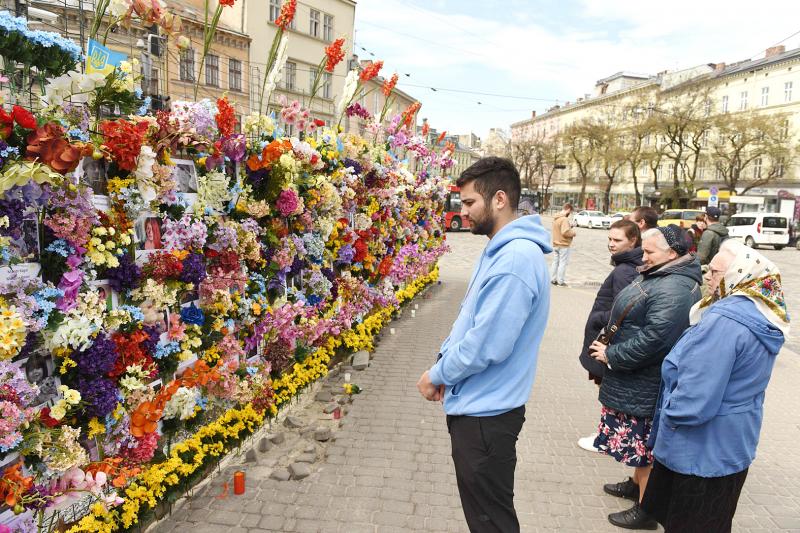The photograph captures a poignant street-level scene of a memorial, featuring an expansive wall adorned with an array of vibrant flowers in shades of purple, blue, yellow, and orange. This floral tribute is interspersed with various pictures and candles, creating a heartfelt homage to the honored individuals. A large row of yellow flowers graces the base of the memorial, while taller orange clusters crown the top. In the foreground, a young man in his 20s with dark hair, wearing a light blue hoodie and pants, stands solemnly with a remorseful expression, examining the memorial. Adjacent to him are three women of varied ages, possibly spanning from their 30s to their 80s, dressed in heavy winter coats and hair bonnets. The setting is a picturesque sidewalk framed by multi-level buildings, trees, and cars, suggesting a small town square, potentially located in Eastern or Central Europe, including regions like the Caucasus, Russia, or Ukraine. The entire scene, bathed in natural light, reflects a collective moment of mourning and remembrance, emphasizing the profound impact of the memorial.